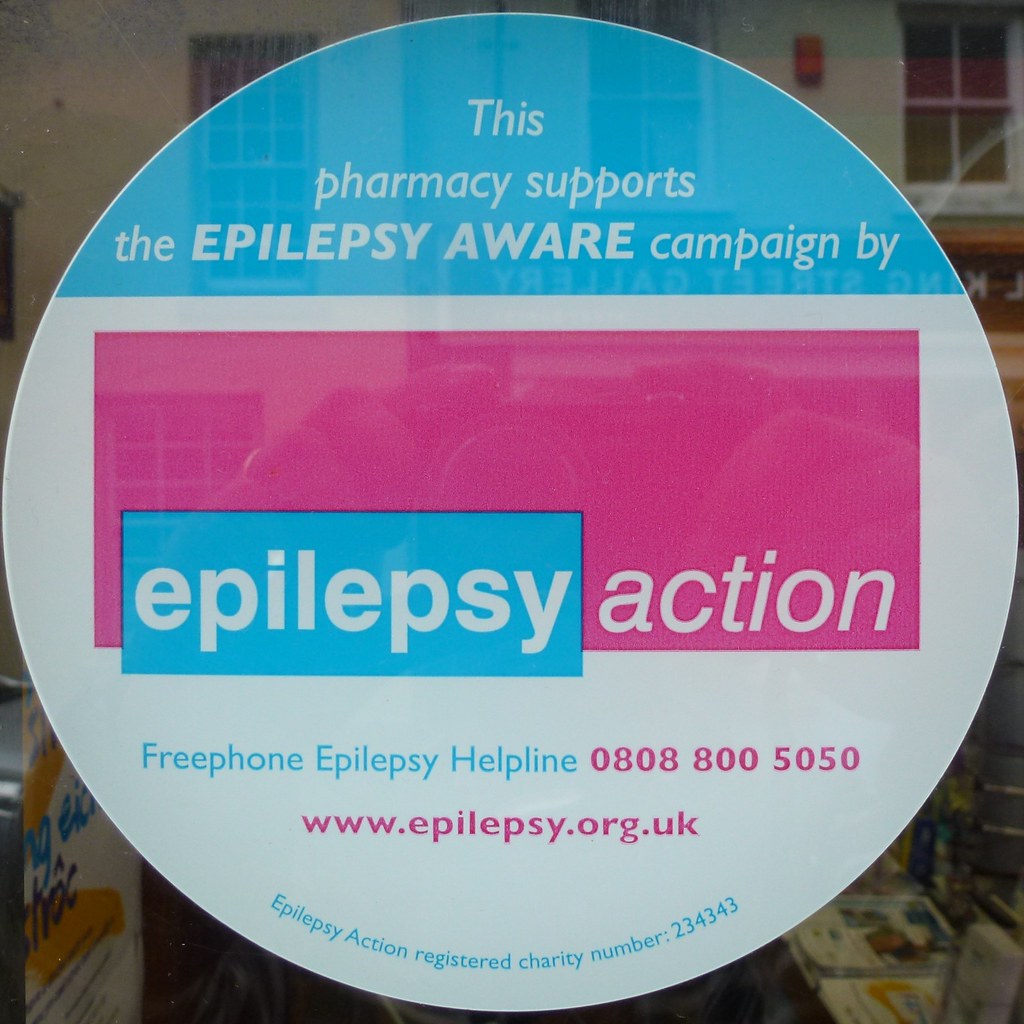The image depicts a circular poster taped to the outside of a pharmacy window, advocating for the Epilepsy Aware campaign by Epilepsy Action. The poster’s top portion displays the text "This pharmacy supports the Epilepsy Aware campaign by" against a blue background. Below this, a prominent pink rectangle encompasses a smaller blue rectangle with the white text "Epilepsy Action." Further down, in pink text, it provides the Free Phone Epilepsy Helpline number "0808 800 5050" and the website "www.epilepsy.org.uk." At the bottom, it lists the Epilepsy Action registered charity number "234343." The text alternates in color between blue and pink, set against a primarily white background. The poster appears to be on an old-fashioned neighborhood pharmacy window in the United Kingdom, with only a dim, partial view of the interior visible.